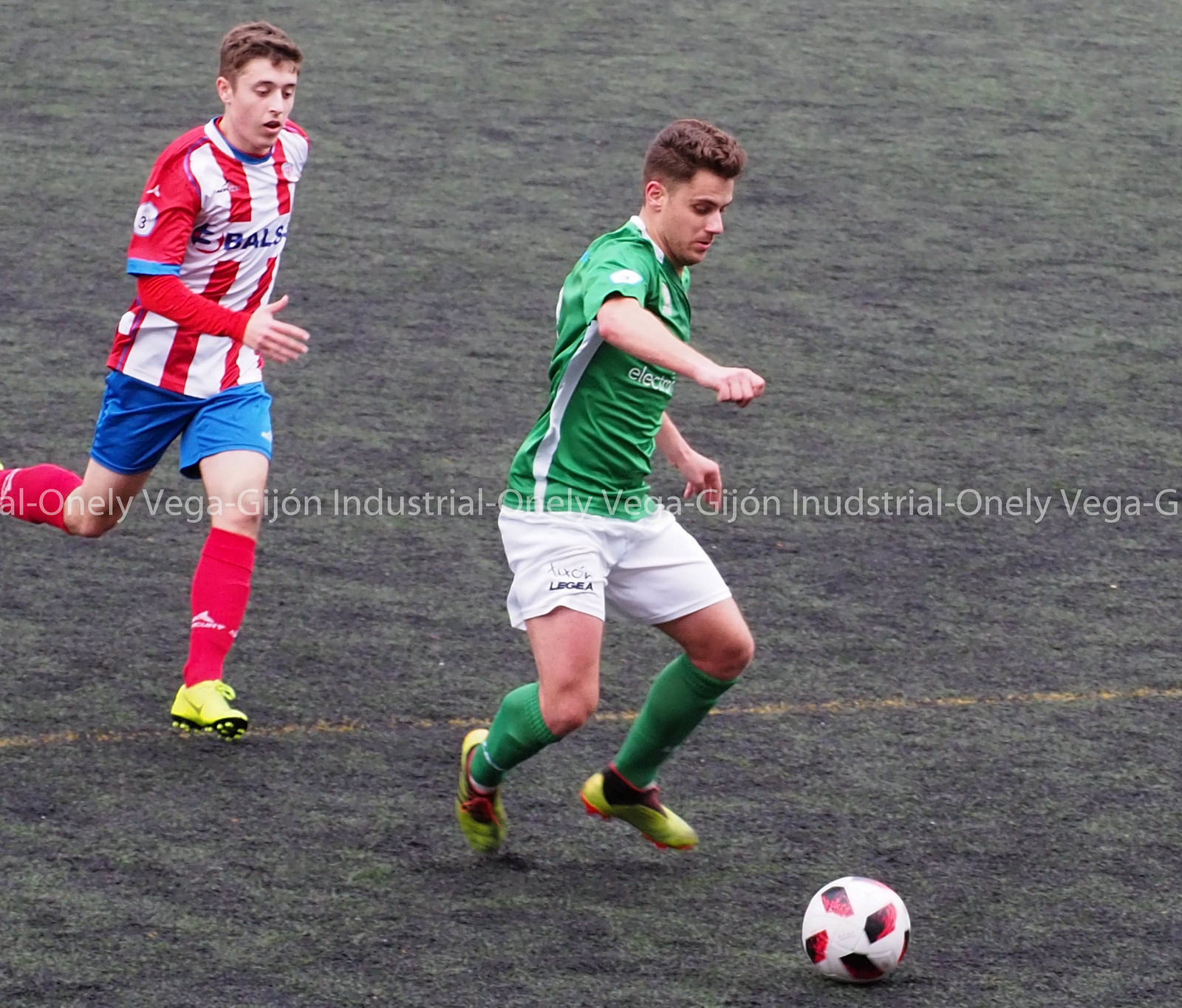In this detailed image, two men are engaged in a soccer game on a dark green astroturf field, marked by a faded yellow line at the bottom. The player at the forefront on the right is about to kick a white soccer ball accented with red and black. He wears a green and white jersey paired with white shorts, green long socks, and fluorescent lemon-and-black boots. This player has short brown hair and appears to be in motion, dribbling the ball. Behind him, another player is chasing. This player, who also has short brown hair, is dressed in a red and white striped short-sleeve jersey over a red long-sleeve shirt, blue shorts, red socks, and bright yellow boots. The text across the screen reads "Vega Dijon Industrial," written in a foreign language.